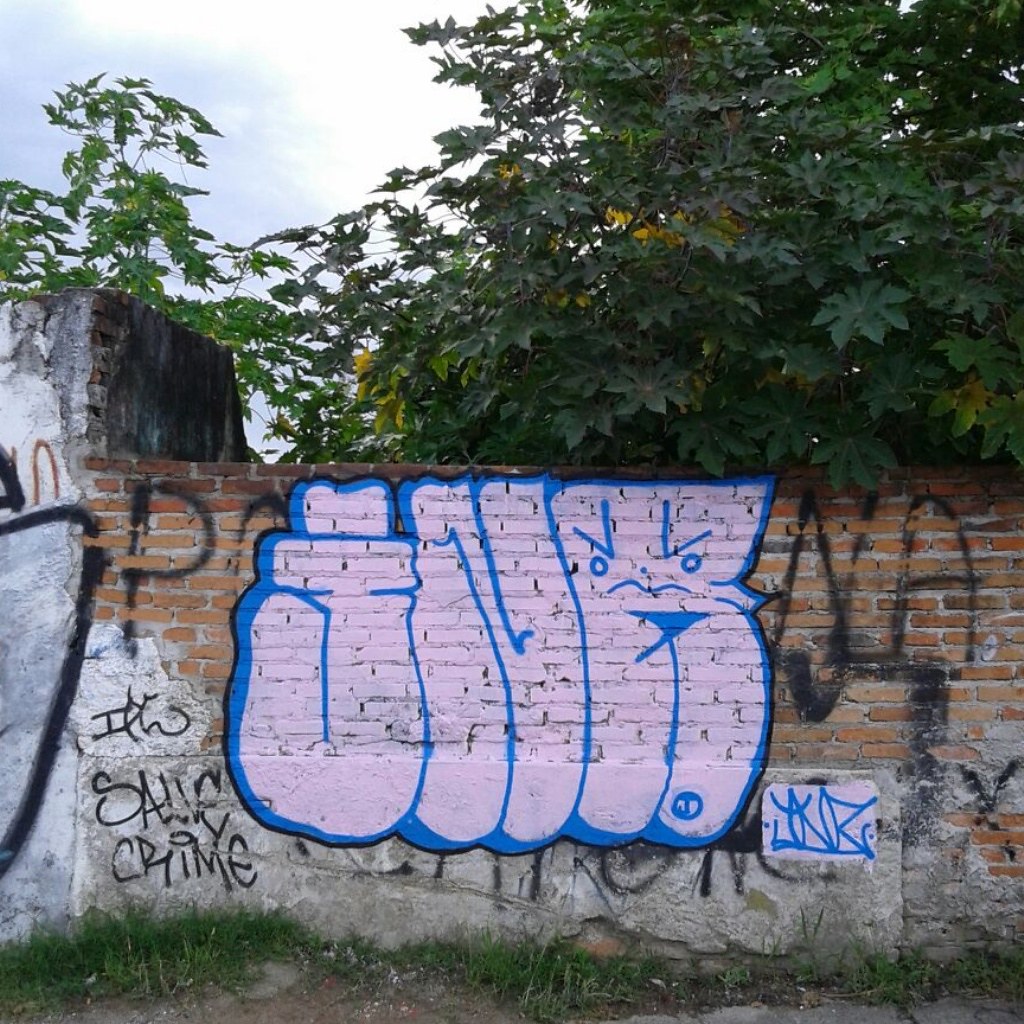The image is a color photograph, captured in portrait orientation, directly facing a short brick wall covered in graffiti. The camera is positioned approximately six feet from the wall, which is about six feet high. The lower half of the wall shows patches of light gray stucco and broken concrete at the base. The ground in front of the wall is a mixture of old, broken concrete, brown dirt, and unruly tufts of grass.

The most prominent piece of graffiti is near the center of the wall, featuring large, vertical letters filled with a light pink color and outlined in blue. To the right of this main graffiti, there is a small pink rectangle with blue initials inside. Additional black graffiti tags are scattered across the upper left, upper right, and along the bottom of the wall.

Above the wall, branches of deciduous trees with dark green and yellow leaves can be seen, framing the scene. A section of light blue sky filled with white clouds peeks through the upper left corner, adding a touch of openness to the otherwise enclosed view.